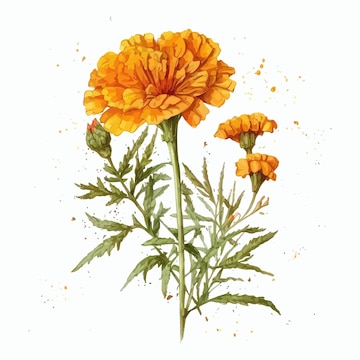The image depicts a detailed, watercolor-style scientific illustration of a bright orange marigold plant. The main flower features a large, dense grouping of vivid, poofy petals atop a sturdy green stem, accompanied by spiky leaves. Extending from the central stem are additional stems bearing green leaves and buds, with two buds on the right beginning to open and a less developed bud on the left. The illustration, evocative of those found in historical botanical catalogues or guidebooks for flower identification, is set against a pristine white background. The background is accented with delicate orange specks, possibly representing floating pollen or paint splatters, adding an artistic touch to the precise botanical rendering.